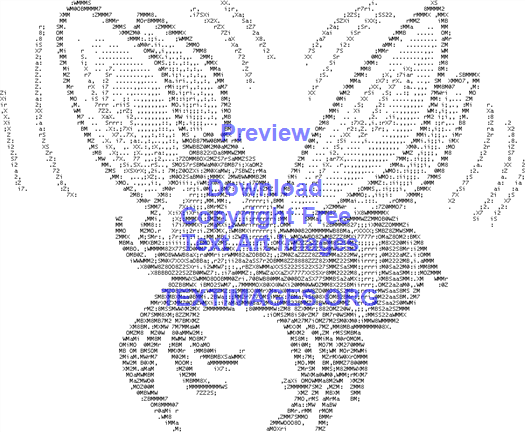The image is an ASCII art representation of a bee, masterfully crafted using various characters such as spaces, numbers, asterisks, and capital letters. The bee features distinct elements like dual wings bordered by motion lines to indicate flapping, and a small stinger at the back, suggesting its identity as a bee rather than a fly. This piece highlights the intricacy of creating motion and form using text characters, a technique popular in earlier digital art. Overlaid on the bee are words in blue: 'preview, download, copyright-free text art images, textimages.org,' indicating the site where this artwork and similar ASCII images can be found. This captivating image serves as both a nostalgic nod to vintage text art and a resource for modern artists seeking unique, downloadable text-based creations.